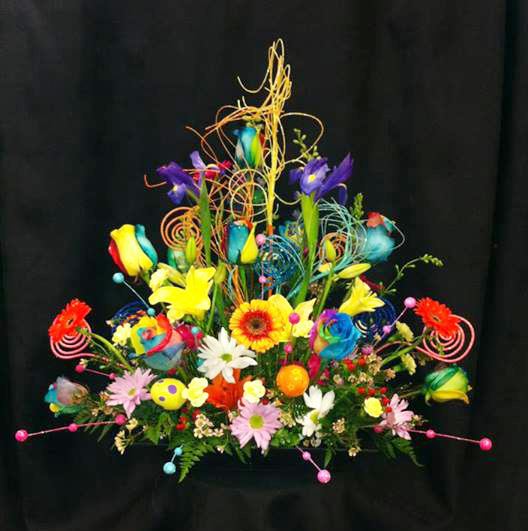The image features a professionally photographed, wildly colorful bouquet set against a black draped background. The carefully arranged floral display is pyramid-shaped, dominated by an array of vividly dyed flowers and enhanced with whimsical decorations. The central composition includes multi-hued roses featuring amalgamations of yellow, blue, and red, alongside bright yellow flowers with striking red centers. Notably, there are vibrant purple irises towards the upper sections and an assortment of white and pink daisies. The bouquet is further filled out with yellow day lilies and fern-like greenery.

Adding to its intricate design, the bouquet is adorned with playful elements such as curlicue painted reeds, beads on wire, and small Easter egg-like balls peeking out from within the arrangement. There are also conspicuous plastic coils and feather-like blue accents interspersed throughout, along with orange and other colored plastic balls that lend a dynamic, almost whimsical quality to the overall display. Despite the apparent tackiness of the artificial components, the bouquet stands out as a vividly colorful and meticulously structured creation, awash in an explosion of colors that pop vividly against the stark black backdrop.